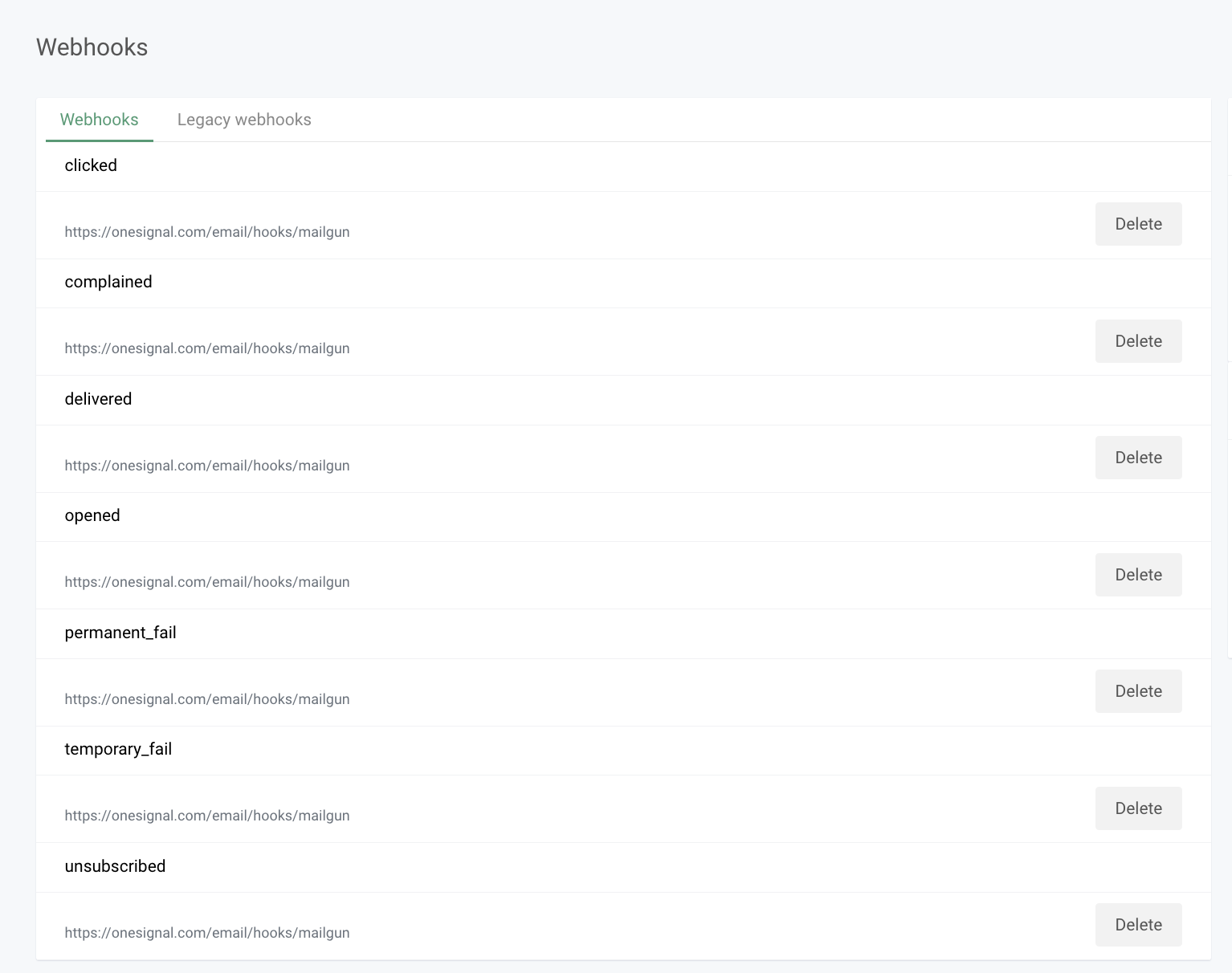Screenshot of a website or application page with a light gray background. In the top left corner, "Webhooks" is displayed in black text. Dominating the page is a large white rectangle. Within this rectangle, two horizontal tabs are positioned in the top left: the first tab, "Webhooks," is highlighted in green text with a green underline indicating it is currently selected; the second tab, "Legacy Webhooks," is in medium gray text and unselected. Beneath the tabs, a thin gray line serves as a separator.

The main section of the white rectangle contains multiple entries, each delineated by thin gray lines. Every entry follows a pattern of bolded text followed by light gray text, ending with a light gray "Delete" button in medium gray text on the far right. The content of the entries lists webhook events and their corresponding URLs, which are all identical, as follows:

1. **clicked** - https://onesignal.com/email/hooks/mailgun - [Delete]
2. **complained** - https://onesignal.com/email/hooks/mailgun - [Delete]
3. **delivered** - https://onesignal.com/email/hooks/mailgun - [Delete]
4. **opened** - https://onesignal.com/email/hooks/mailgun - [Delete]
5. **permanent_fail** - https://onesignal.com/email/hooks/mailgun - [Delete]
6. **temporary_fail** - https://onesignal.com/email/hooks/mailgun - [Delete]
7. **unsubscribed** - https://onesignal.com/email/hooks/mailgun - [Delete]